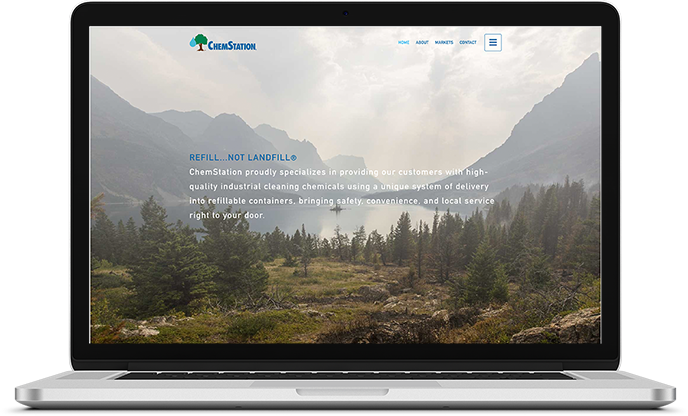The image features an open laptop showcasing a striking juxtaposition of modern technology and natural beauty. The laptop's keyboard is black, contrasting with its silver or light gray housing that surrounds the keys and extends to the device's sides. The monitor bezel is black, framing an awe-inspiring screen display of an outdoor landscape. In the background, towering mountaintops stretch skyward, while below, a lush valley blanketed with pine trees and verdant grass unfolds. A serene lake glimmers in the distance, adding to the picturesque scene.

In the upper left corner of the screen, the blue text "Chem Station" is paired with an illustrated tree, introducing the focal point of the image. Just below that, more blue text reads, "refill, not landfill," emphasizing the eco-friendly message. In white text beneath that, a concise yet informative tagline explains, "Chem Station proudly specializes in providing our customers with high-quality industrial cleaning chemicals, using a unique system of delivery into refillable containers, bringing safety, convenience, and local service right to your door."